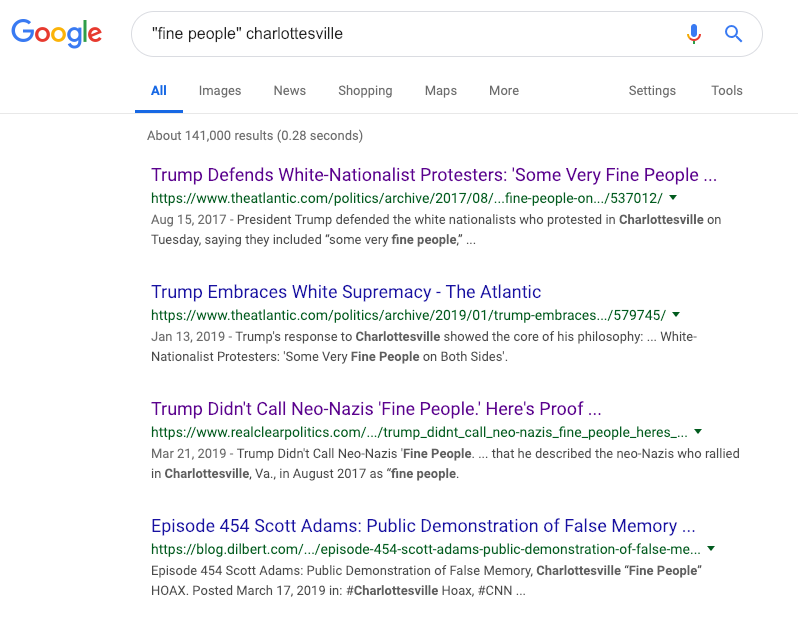**Descriptive Caption:**

The image displays a web page showcasing Google search results. At the top-left corner is the Google logo. Within the search box, the query "find people Charlottesville" is entered. Adjacent to the right of the search box, there's a microphone icon with a blue top and red bottom, alongside a blue magnifying glass icon. 

Below the search box, the "All" tab is highlighted in blue and underlined, indicating the active search filter. Other available options include Images, News, Shopping, Maps, More, Settings, and Tools shaded in gray. A thin gray line separates these tabs from the search results.

The search results indicate approximately 141,000 results returned in 0.28 seconds. The first and third search results appear in purple text, signifying that they have been read. The first result headline reads, "Trump defends white nationalist protesters, some very fine people," linking to an article from The Atlantic dated August 15, 2017.

The second result headline is "Trump embraces white supremacy – The Atlantic," with a link to another article from the same publication dated January 13, 2019. The third result, also in purple text, states, "Trump did not call neo-Nazis fine people, here's proof," from RealClearPolitics, dated March 21, 2019.

The fourth result, which appears in blue and has not been read, is titled "Episode 454, Scott Adams, public demonstration of false memory," from the Dilbert blog.